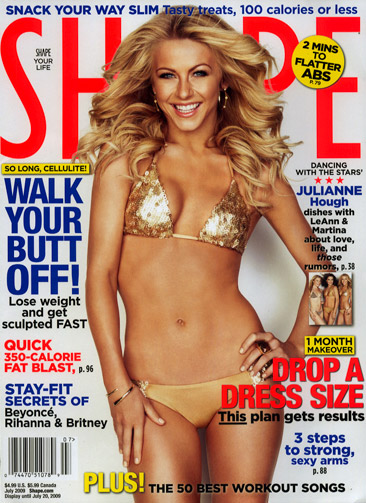A vivid magazine cover for Shape Magazine features Julianne Hough prominently displayed in the center, radiating in a golden bikini. The cover is peppered with vibrant colors including gray, blue, orange, yellow, black, white, and tan. Various enticing headlines surround her with enticing fitness advice and celebrity insights. At the very top, bold text invites readers to "Snack your way slim with tasty treats 100 calories or less." Directly beside Julianne, captions boast quick weight loss regimes such as "Walk your butt off, lose weight, and get sculpted fast" and "Quick 350 calorie fat blast." On the left side, viewers are teased with "So long cellulite" and an exclusive featuring Julianne herself, "Dancing with the Stars' Julianne Hough dishes with Leanna Martina about love life and those rumors – page 38." Additional highlights include "Stay fit secrets of Beyonce, Rihanna, and Britney," a "One-month makeover part," steps to "Drop a dress size," a plain but effective approach for "Three steps to strong sexy arms," and a list of the "50 best workout songs," promising a trove of practical tips and motivational reads within.